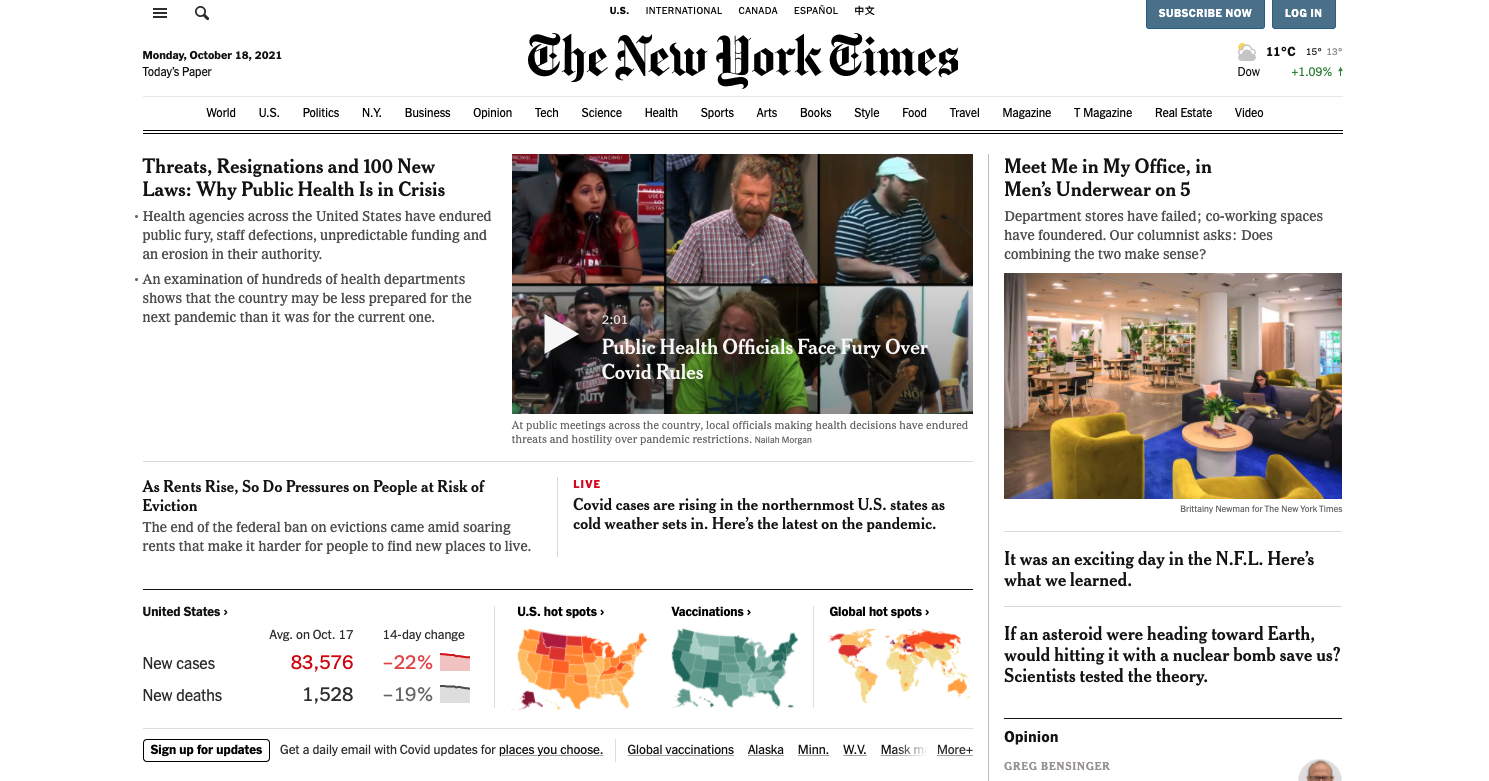The webpage from the New York Times features its iconic name and font prominently displayed in black at the top, set against a white background. Below the header, there are various sections of the newspaper that users can click on.

On the left side of the page, the headlines read "Threat of Resignation and 100 New Laws." Adjacent to this, there is a visual of six individuals grouped together in a rectangular photo with the caption, "Public Health Officials Face Fury Over COVID Rules." 

To the right, there's an article titled "Meet Me in My Office: In Men's Underwear on Fridays" accompanied by a few preview sentences. Directly beneath this, another photograph is displayed.

Further down the page on the left, there are brief summaries of two more subjects. Just beneath these, a weather map is displayed, labeled "United States," but it appears to present COVID-19 data instead. 

Adjacent to this are three maps visualizing COVID-19 related statistics: two maps of the United States showing hotspots and vaccination coverage in varying colors, and one global map indicating international hotspots, captioned "Global Hotspots." 

Towards the end of the page, there's a call-to-action for readers to sign up for daily email updates on COVID-19, tailored to the locations of their choice. Below this, statistics show that new COVID-19 cases number 83,576, a 22% decrease over the past 14 days, underscoring the assumption that the data is related to COVID-19 updates.